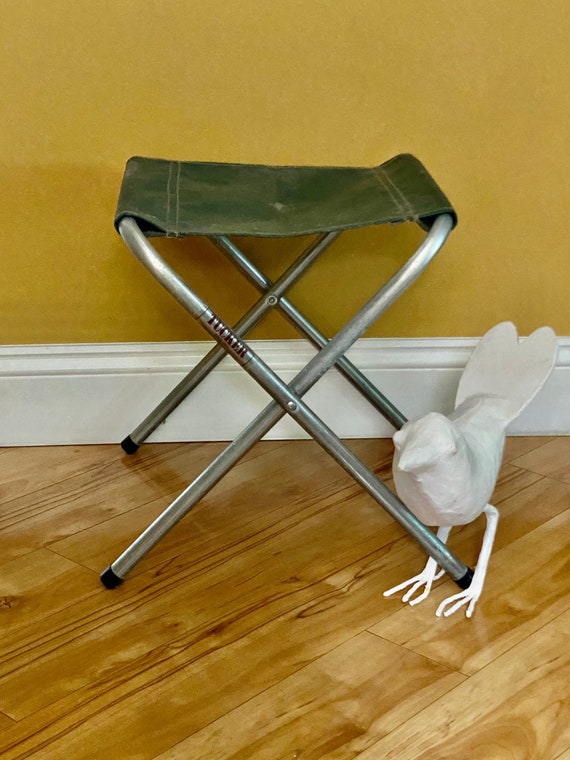This image features a fold-out stool with an olive green canvas seat and a metal frame composed of U-shaped, aluminum or chrome bars that cross in an X-pattern at both the front and back. The stool is fully set up on a polished, shiny wooden floor with planks oriented diagonally from the bottom left to the upper right. The backdrop includes a white baseboard and mustard yellow walls with a gold-like appearance. To the right of the stool stands a white, stylized bird sculpture with indistinguishable features and a heart-shaped tail that extends above the baseboard. The bird's beak points forward, and its right leg is positioned behind one of the stool's front legs, creating a slightly tucked-in look. The word "Tucker" is visible on one of the stool's metal bars.